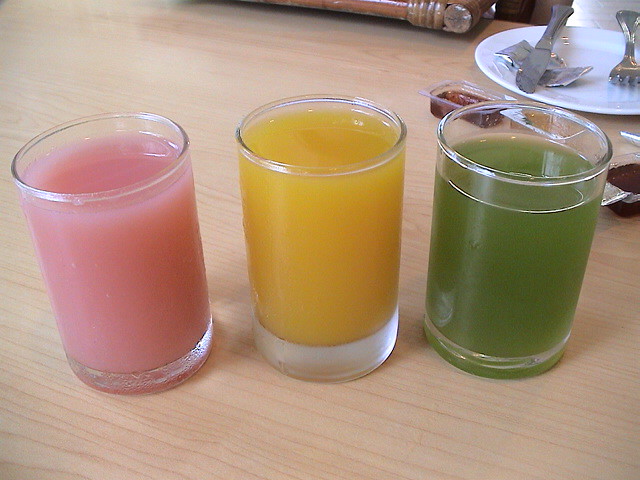In the photo, a light-colored wooden table features three clear glasses, each filled almost to the brim with opaque liquids of different colors. The glass on the left contains a pink liquid, the middle glass has an orange liquid, and the glass on the right holds a green liquid. In the background to the top right, a white plate with a silver fork and knife can be seen. Surrounding the plate, there are small open containers of strawberry jelly, with their foil wrappers still on the plate. This detailed breakfast setting appears to be in a restaurant booth, with no people or text visible in the image.